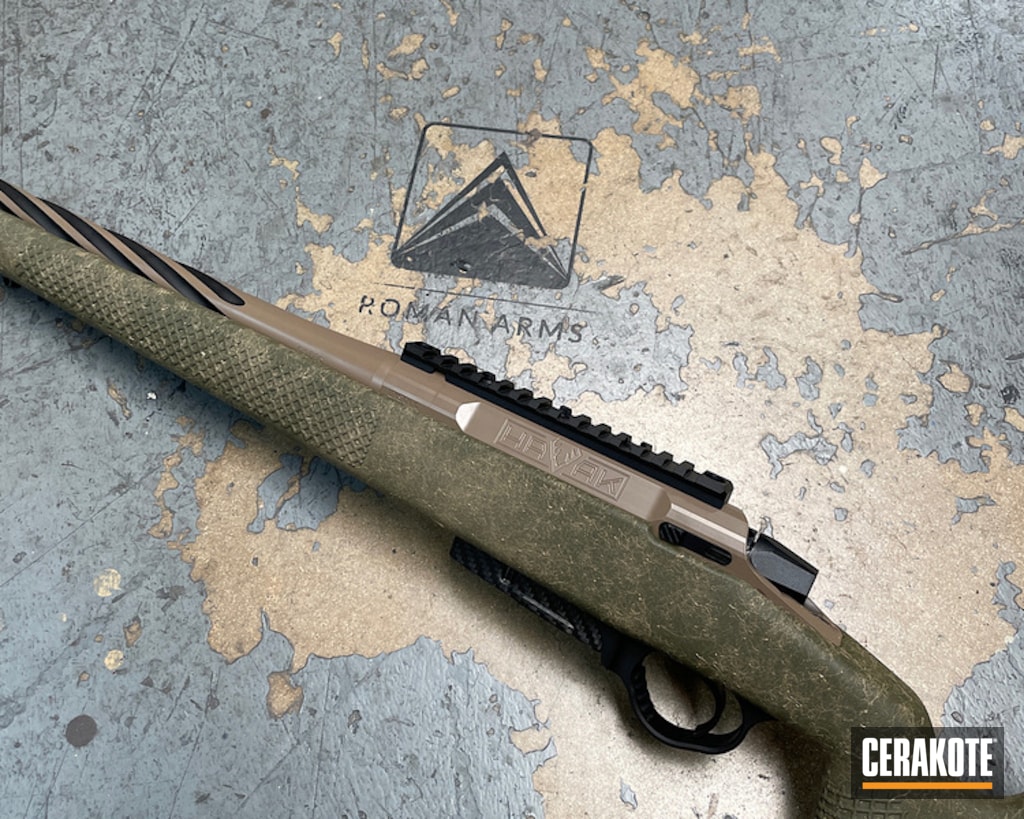This image features an antique firearm, likely a rifle, displayed on a scratched and chipped gray-painted surface with beige undertones. The rifle, which is partially visible without the butt or front end, exhibits a green patina and a snake-like scaled pattern toward the front. The firearm's long brownish sight range spans the top, and the black trigger mechanism is clearly visible underneath. In the backdrop, a rectangular, black-outlined frame is situated near the center top, containing a series of stacked black and clear triangles, resembling pyramids, and labeled "Roman Arms" in bold, uppercase letters. Additionally, a black rectangle with "CERAKOTE" in white uppercase letters and a horizontal orange line beneath it is positioned in the bottom right corner of the image. The background also shows evidence of white paint splatters and extensive scratches, enhancing the antique and worn appearance of the setting.